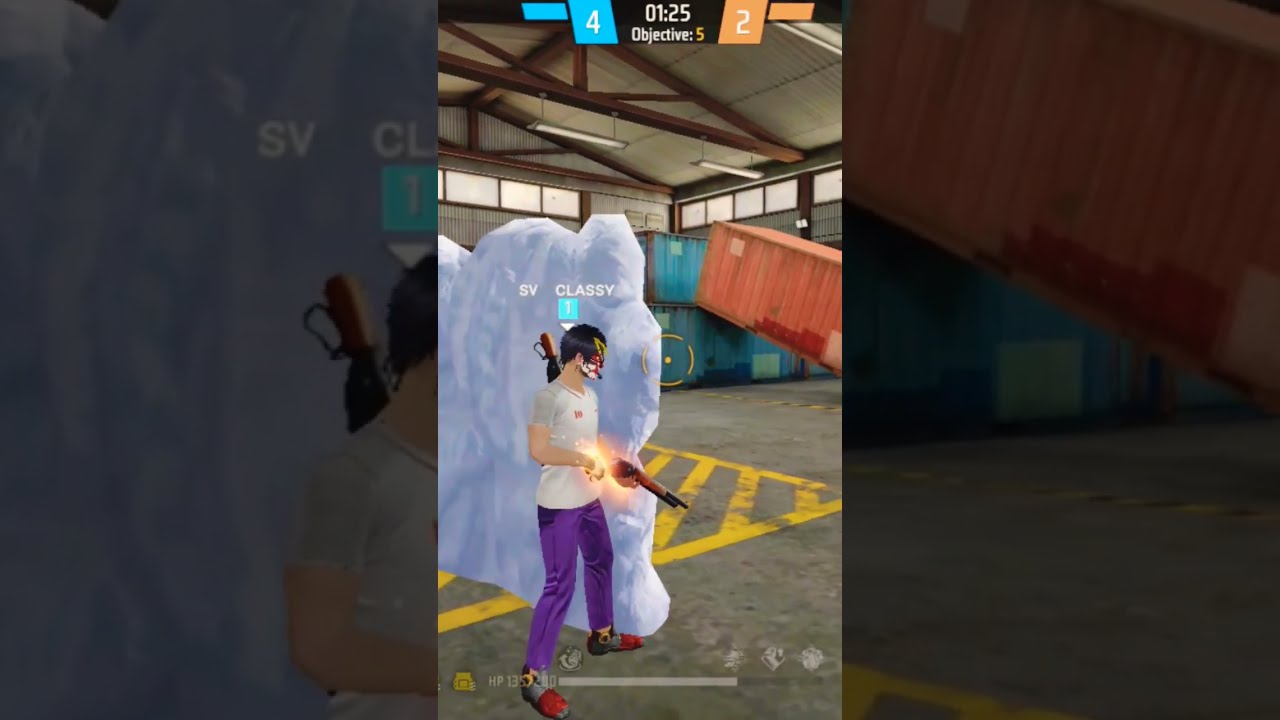This image is divided into three vertical sections, with the left and right sections showing darkened close-ups of the central section. The central section is a screenshot from a video game set inside a large warehouse. The character in the center is wearing purple pants, a white short-sleeved t-shirt, and gray and red shoes. They have a mask with red and yellow colors on their face. The character is armed with a gun in their left hand and a second gun on their back, while their right hand appears to be glowing slightly. They are positioned behind a wall-like structure that resembles white pillows or possibly ice. The warehouse setting features a gray cement floor with yellow patterns, and in the distant background, there are blue and orange metallic containers. Above the character, at the top of the screen, there are game stats displayed with the number four in blue on the left and the number two in a peach block on the right. Below the stats, in a black block with white writing, it reads "1.25 objective 5." Additional stats can be seen at the bottom of the screen. Positioned above the character is some text that reads "SV Classy 01."